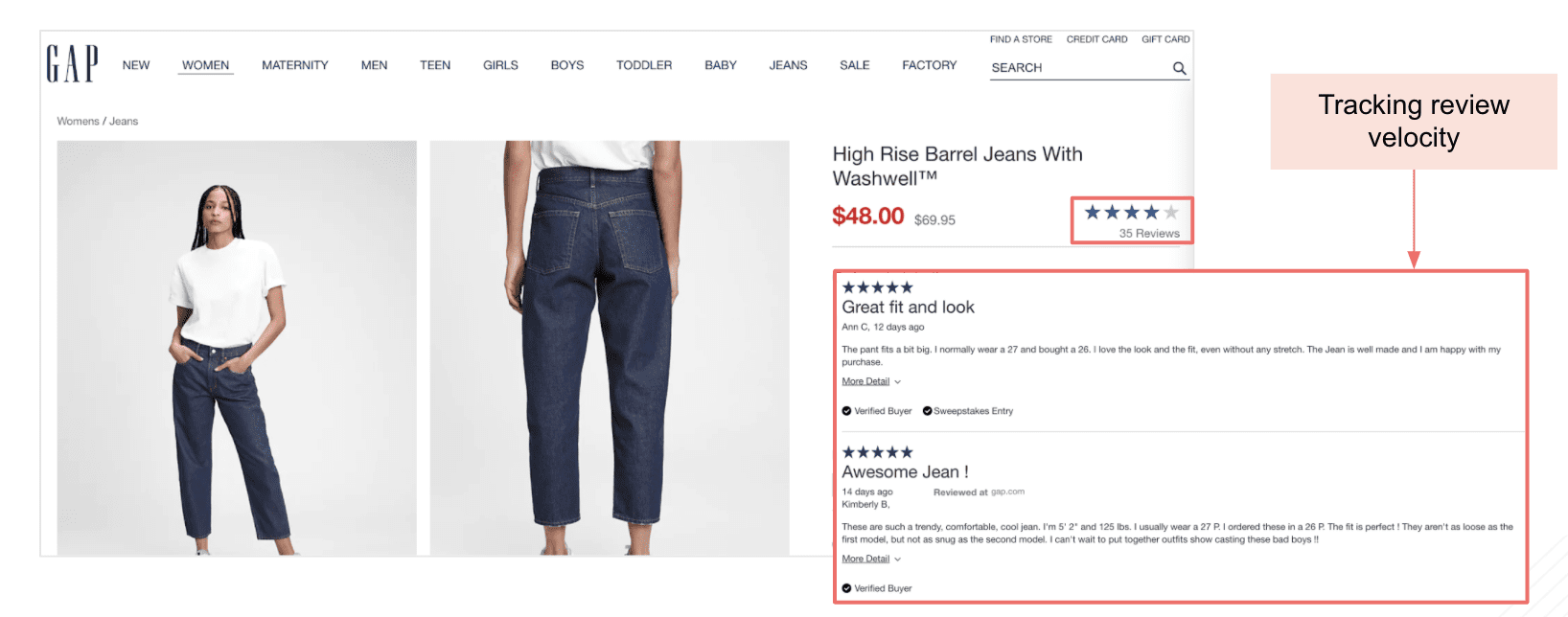This is a detailed screenshot from the GAP website featuring a light gray border around the edges. At the top, the menu lists categories such as GAP, New Women, Maternity, Men, Teens, Girls, Boys, Toddlers, Babies, Jeans, Sale, and Factory. A search bar is positioned to the right. 

Below the menu, there are two pictures. One shows a Black woman modeling a casual outfit, specifically a white t-shirt paired with loose-fitting jeans. The product description identifies these jeans as "High-Rise Belgian" with "Washwell" technology, priced at $48. The item has received a solid rating of four stars.

Adjacent to the product image, a pink rectangle displays the text "Track and Review Velocity" in black letters, accompanied by an arrow pointing towards a red (or pink) colored box. Inside this box, against a white background, are various customer reviews. The top review gives the jeans a perfect score of five out of five stars and describes them as having a "Great fit and look." The second review also awards the jeans five out of five stars, noting simply, "Awesome jeans."